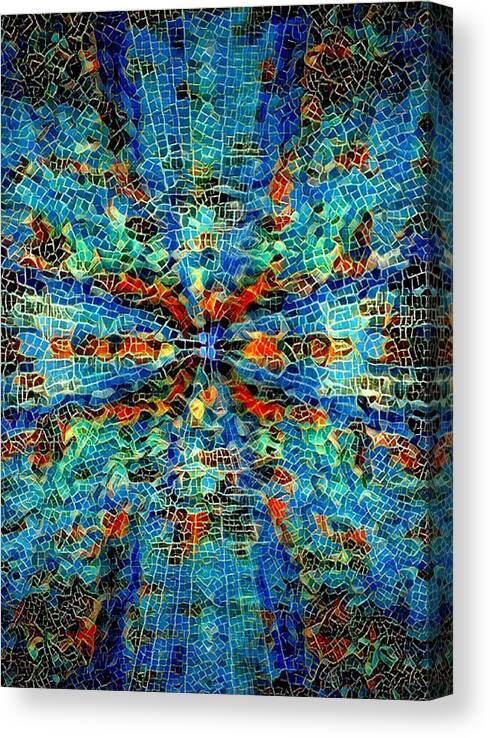This is a detailed description of an abstract painting represented digitally on a rectangular canvas, framed against a solid white background that casts a light gray shadow to the right and bottom, giving it a 3D appearance. The painting, which tilts slightly towards the left, features a vibrant and colorful mosaic or stained glass style. Predominantly, the artwork uses bright hues of blue and green, punctuated by four red lines radiating from the center, forming a flower-like pattern. These radiant lines are surrounded by blue and green mosaic tiles, all edged with a light yellow outline, enhancing their separation and adding depth. The canvas corners transition into darker tones, blending blacks with specks of blue, red, green, and other colors of the rainbow, creating an effect that both grounds the piece and makes the luminous center stand out. The artwork, devoid of any text, combines elements reminiscent of a Gothic stained glass window, exuding a timeless quality that makes it suitable both for a modern home setting or an art collector's portfolio.